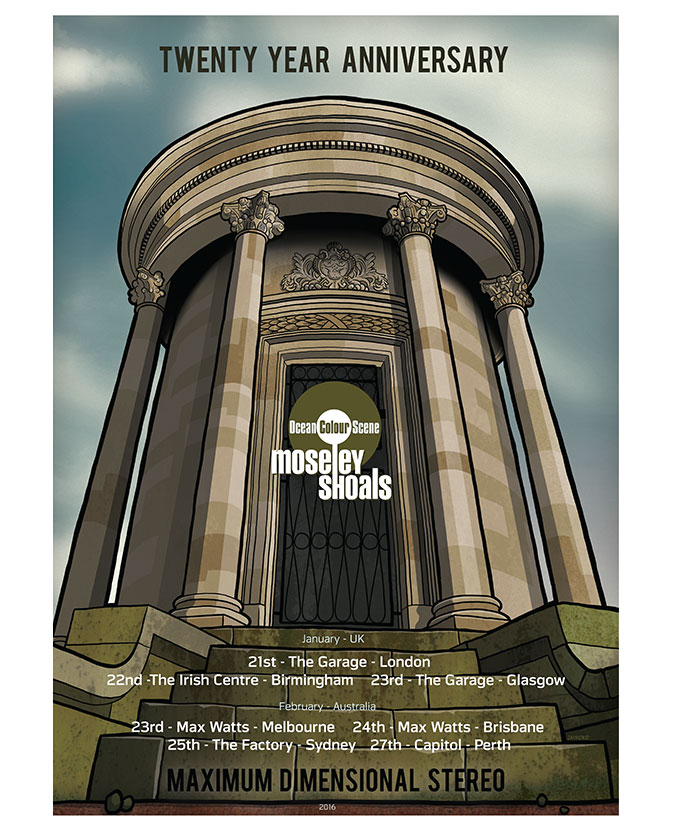The image showcases a graphic advertisement for an event celebrating the 20-year anniversary of the band Ocean Color Scene's album "Moseley Shoals." The background features a blue sky with a few clouds, seemingly taking up most of the picture, and is bordered in blue along the top and sides. 

Central to the image is a large, imposing structure resembling a mausoleum or memorial with four tall, circular beams and five steps leading up to it. The building has a big door adorned with the Ocean Color Scene logo, which is white with an olive green circle and text. 

At the top of the image, in black text, it reads "20 Year Anniversary." Below this, the event details are laid out in white text:

- January UK: 
    - 21st: The Garage, London
    - 22nd: The Irish Centre, Birmingham
    - 23rd: The Garage, Glasgow

- February Australia: 
    - 23rd: Max Watts, Melbourne
    - 24th: Max Watts, Brisbane
    - 25th: The Factory, Sydney
    - 27th: The Capital, Perth

At the very bottom of the steps, in black text, it states "Maximum Dimensional Stereo."